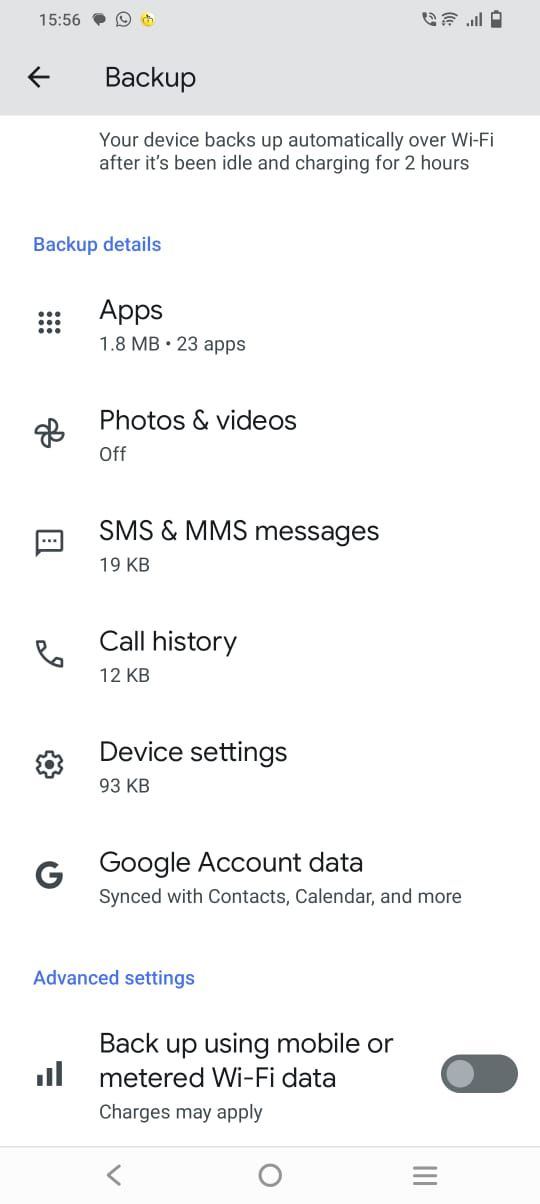This screenshot, captured on a smartphone at 15:56, showcases the device's screen displaying the "Backup" settings interface. In the upper-right corner of the screen, icons for a messaging app and a calling app are visible. To the right, the phone's status icons indicate that Wi-Fi is connected, the signal strength is good, and the battery level is approximately at 50%.

At the top center of the screen, the title "Backup" is displayed with a left-pointing arrow beside it. Below this, a message explains that the device automatically backs up over Wi-Fi after being idle and charging for two hours. This text is in a grayish-black font, while the "Backup details" section title beneath it is in blue font.

The "Backup details" section itemizes various categories and their respective storage allocations and statuses:
- Apps: 1.8 MB, covering 23 apps
- Photos and Videos: Off
- SMS and MMS Messages: 19 KB
- Call History: 12 KB
- Device Settings: 93 KB
- Google Account Data: Synced, including contacts, calendar, and more

Beneath this section, the "Advanced settings" link is displayed in blue font. Following that, an option to "Backup using mobile or metered Wi-Fi data" is listed, with a caution that charges may apply. The toggle switch for this option is currently turned off, indicated by the grayed-out circle positioned to the left.

At the bottom of the screen, classic navigation icons are presented: a left-pointing arrow for back, a circular home button, and a three-line menu button for more options.